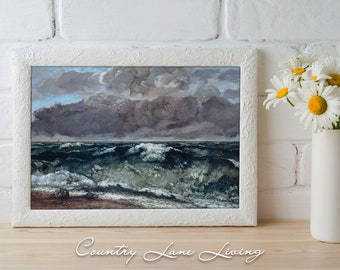The image features a detailed scene with several elements arranged artfully. Dominating the background is a white brick wall that has been painted over, providing a clean and uniform surface. Against this wall, more to the left in the composition, rests a picture with a rough-textured white frame. The painting inside the frame depicts a turbulent ocean wave in dark, almost black blue hues, crashing against a sandy shore on the bottom left. Above the waves are heavy, thick gray clouds interspersed with small patches of blue sky, adding to the dramatic atmosphere of the scene. On the surface beneath the picture, made of light brown wood, cursive writing spells out "Country Lane Living," adding a quaint and rustic touch. To the right of the picture frame stands a smooth, cylindrical white vase containing several white flowers with striking yellow-orange centers, providing a contrast to the darker tones of the painting and adding a fresh, brightening element to the overall composition.